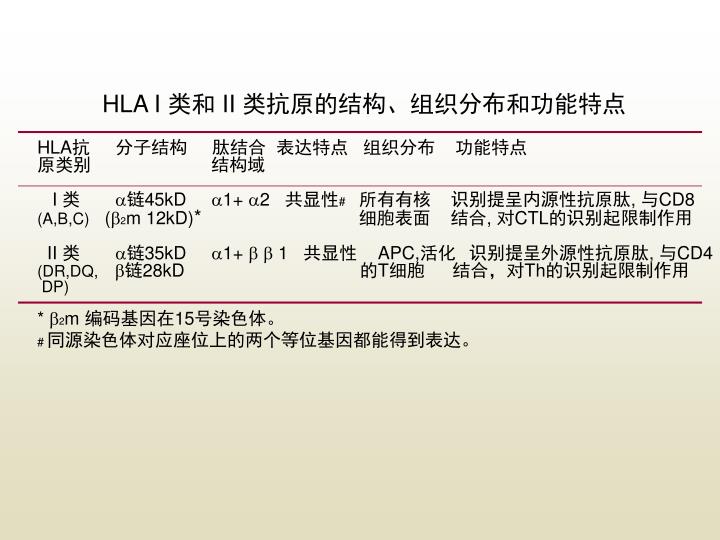The image is a detailed depiction featuring a white background that gradually transitions to an off-white hue lower down. Across the top is a prominent title in Western characters: "HLA I," followed by additional text in Chinese or Japanese characters. The layout is structured with six rows of information, each separated by red lines. Specifically, the first bold red line is located just beneath the title, another red line divides the middle of the image, and a fainter, lighter red line is situated closer to the top, near the first red line. These sections contain a mixture of the Asian characters and Western alphabet letters, along with potential mathematical formulas, indicating that the text may relate to a mathematical or educational context.